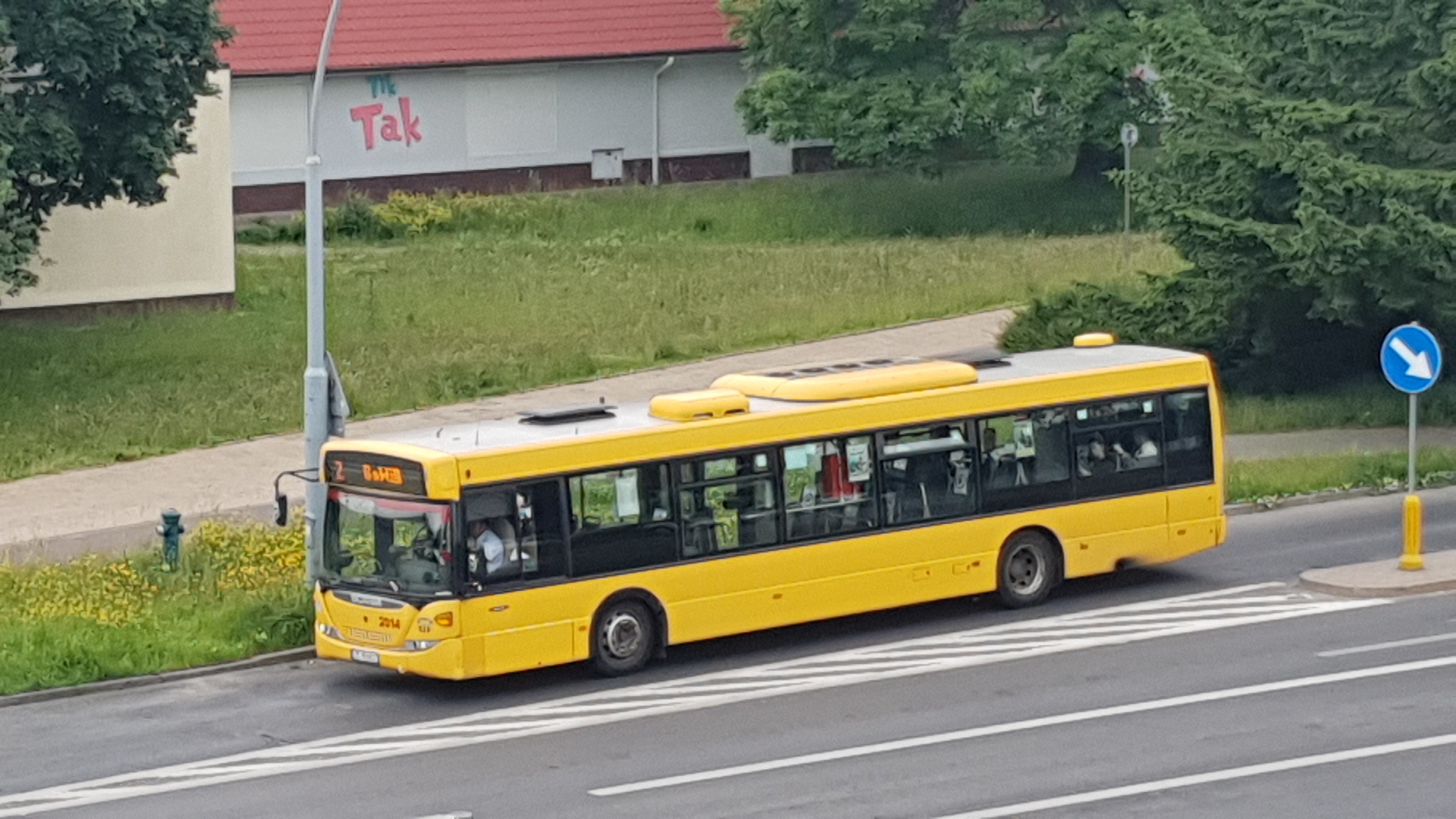The image depicts a vibrant street scene centered around a long yellow city bus with large windows, through which the driver in a white shirt is visible. The bus, adorned with a digital display on its upper front section, traverses a road marked with white broken lines. Adjacent to the bus stands a tall street lamp and a small green fire hydrant emerging from a grassy patch dotted with yellow flowers. This grassy area transitions into a sidewalk that stretches horizontally across the scene. Beyond the sidewalk, another field of taller grass leads to a picturesque backdrop featuring trees and a prominent white building with a pink roof. The building has the letters "TAK" emblazoned on its side in bold pink lettering.